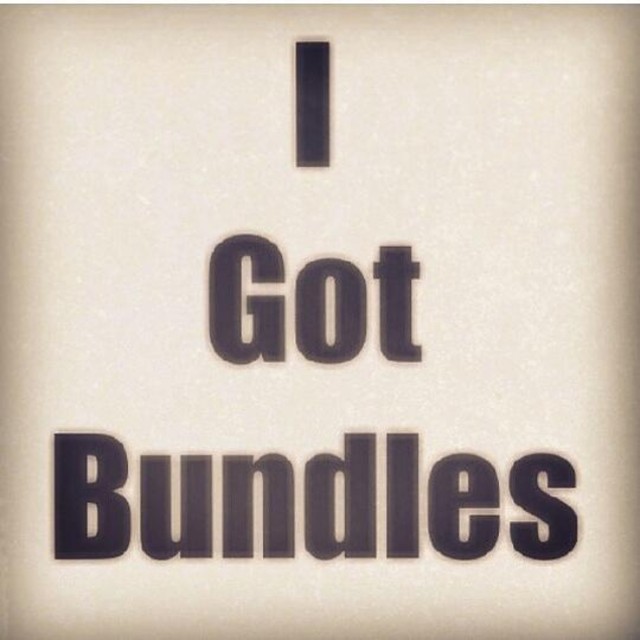The image is a low-resolution, heavily pixelated and artifacted screen grab, possibly advertising something. It features a simple and minimalistic design with a central tannish or off-white background that darkens towards the edges, creating a faded black, vignette-like effect. In the center, there are three lines of bold black text, each word on a separate line, reading: "I" on the top line, "got" on the middle line, and "bundles" on the bottom line. The letters appear somewhat hazy and distorted due to the poor image quality, emphasizing its simplistic and straightforward nature.